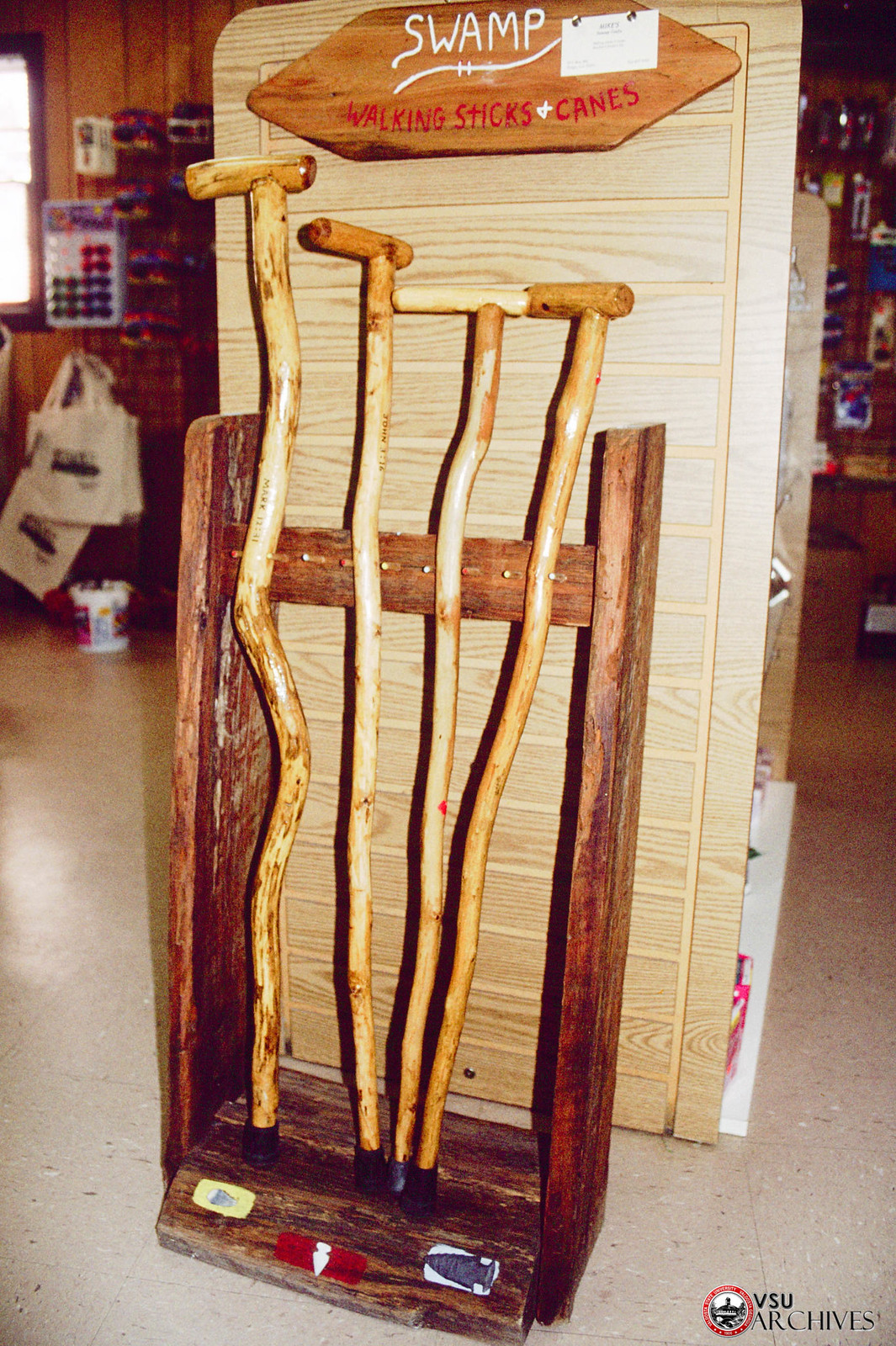The image captures a rustic, indoor store display featuring a small wooden rack holding four handmade canes. These canes, crafted from light brown, twisted natural sticks, exhibit a roughed and aged appearance and are fitted with rubber mounts at their bottoms. The rack itself, dark-stained and weathered, includes decorative elements such as arrowhead stickers at its base. Positioned at the end of an aisle, the rack bears a football-shaped wooden sign above it, inscribed with "SWAMP" in white and "WALKING STICKS AND CANes" in red lettering. Behind the main display, there's a wooden shelf stocked with various items, including tote bags and a countertop display of sunglasses and multicolored products. On the right-hand side, additional items hang from a wall display, while the floor appears to be gray, possibly tile or linoleum. In the bottom right corner, a circular logo with the text "VSU Archives" in black letters is visible, adding a formal touch to the scene that evokes the ambiance of an old-fashioned country sundry store.